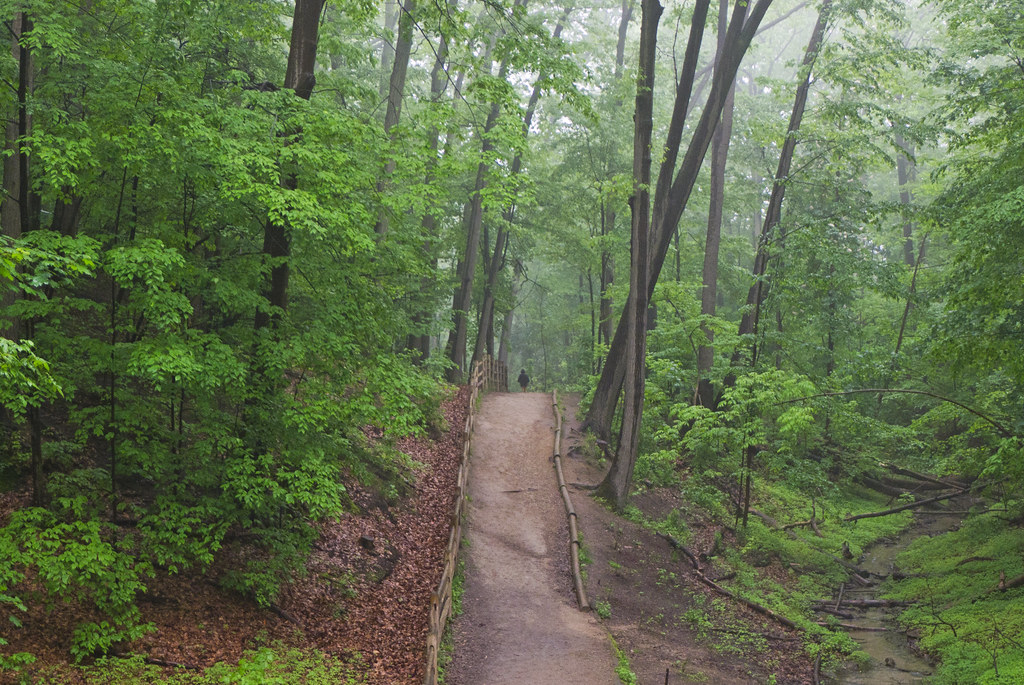A tranquil, misty forest scene unfolds with a well-defined hiking trail at its center, bordered on the left by a wooden split rail fence and by logs on the right. The smooth, brown trail ascends a gentle hill, with the distant silhouette of a person in a dark jacket and lighter pants just cresting the peak, appearing as a tiny dark figure. The forest is lush and green, with tall, thin trees creating a dense canopy, and there's a small, meandering white creek running along the far right side of the image, surrounded by mossy greenery and fallen trees. The ground appears damp, likely from recent rain or lingering fog, enhancing the serene and peaceful ambiance.